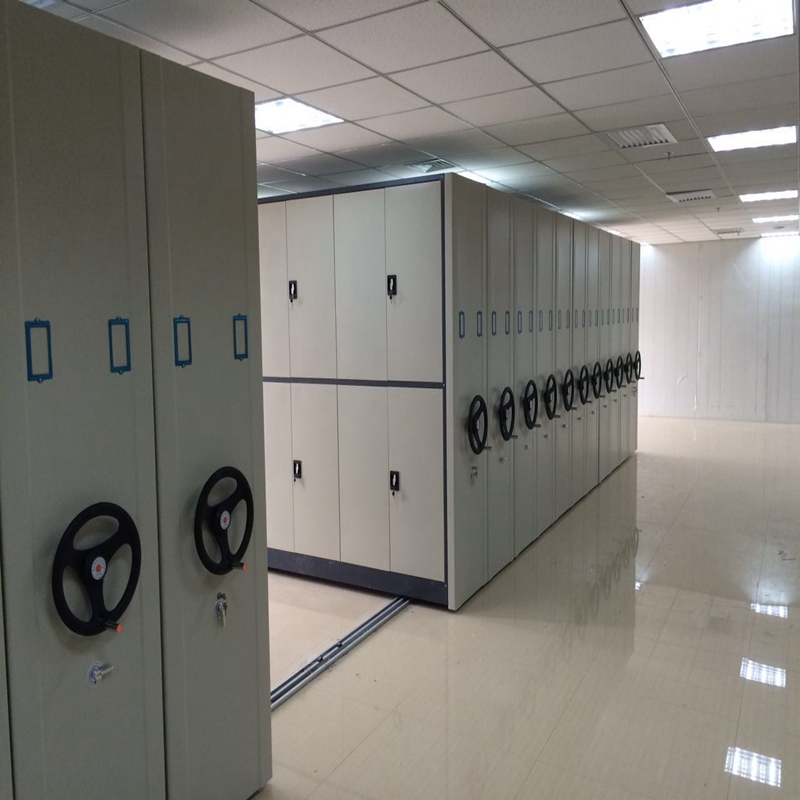The image depicts a highly organized archive room, featuring multiple rows of off-white, secure vault-like filing cabinets. These cabinets, which are designed to store large volumes of files, photos, or newspaper clippings, are equipped with black hand cranks that allow users to move them along a metal railing system on the floor. The well-lit room has a pristine, white ceiling adorned with square lights and vents, enhancing the bright white ambiance. The shiny, waxed tan floor reflects the ceiling, adding to the room’s clean and orderly appearance.